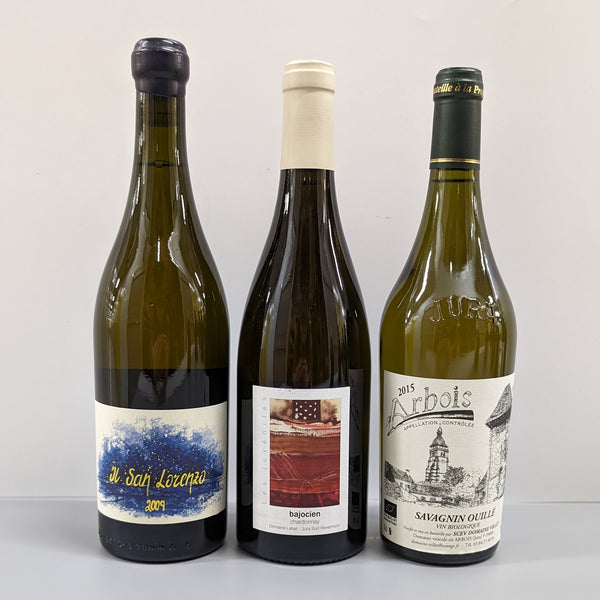The image depicts three wine bottles standing side by side against a plain backdrop. The first bottle on the left is an olive green glass with a black foil covering the cork. It features a blue, white, and yellow label that reads "M. San Lorenzo, 2009." The second bottle, in the middle, has a dark green—almost black—hue with a white foil on the cork. Its white label, adorned with reddish-brown details, identifies it as "Bajocin, Chardonnay." The third bottle on the right is another olive green glass, topped with a green foil and gold lettering. The label is white with a black and white illustration of buildings in a countryside setting, reading "2015 Arbois, Appellation," followed by partially legible text starting with "Savagninouille." The focus of the photograph is exclusively on these three distinct wine bottles.